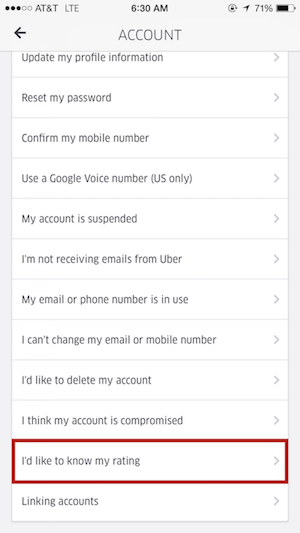The image displays a screenshot from a cell phone, which is connected to the AT&T network with LTE service. The status bar at the top indicates the time is 6:30 a.m., the battery level is at 71%, and several additional icons are visible. Below the status bar, the screen title "ACCOUNT" is displayed in all capital letters and a grayish font, with a left-facing arrow in the upper left corner. 

The screen lists various account-related options in a vertical menu format:
1. **Update My Profile Information**
2. **Reset My Password**
3. **Confirm My Mobile Number**
4. **Use a Google Voice Number (US only)**
5. **My Account Is Suspended**
6. **I'm Not Receiving Emails from Uber**
7. **My Email or Phone Number Is in Use**
8. **I Can't Change My Email or Mobile Number**
9. **I'd Like to Delete My Account**
10. **I Think My Account Is Compromised**
11. **I'd Like to Know My Rating** (this option is highlighted with a red rectangle border)
12. **Linking Accounts**

The detailed visual representation of various options suggests this image is likely from a user settings section within an app, providing multiple avenues for account management and troubleshooting.